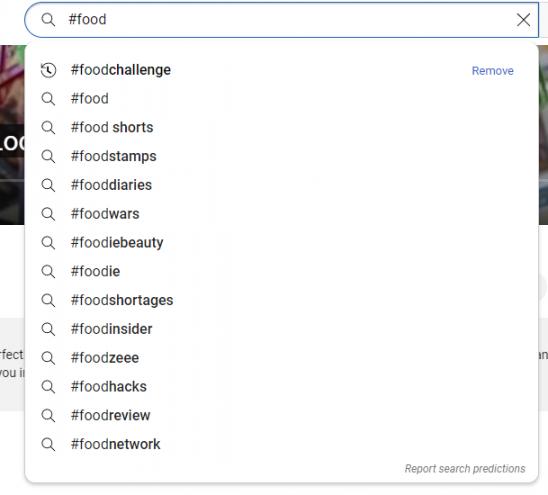A screenshot capturing a search bar at the top with "#food" entered, flanked by a small 'X' on the far right, indicating the option to clear the search term. Below are a series of dropdown search suggestions populated from previous interactions and common queries, each preceded by a hashtag symbol and a search icon. Notable suggestions include "#foodchallenge," "foodshorts," "foodstamps," "fooddiaries," "foodwars," "foodiebeauty," "foodshortages," "foodinsider," and "foodnetwork." On the bottom right corner, there's an option to "Report search predictions." Faintly visible in the background are the blurred edges of an image with partial text on the bottom left spelling "F-E-C-T-O-U-L," and on the bottom right, the letter 'N'.